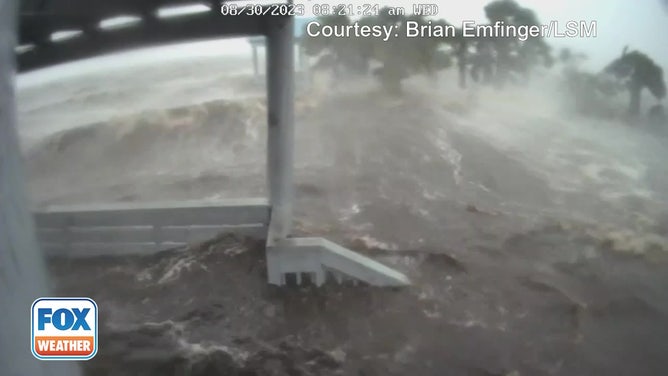The image appears to be a screenshot from a video, likely taken from a Fox Weather broadcast, as indicated by the "Fox Weather" logo in blue at the bottom left corner. The scene depicts a severe flood, possibly due to a hurricane or storm surge. The floodwaters, which are muddy and turbulent with white froth, engulf what looks like the porch of a house. A steel pillar in the center goes down to what appears to be part of a deck wall, with horizontal wood planks extending to the left and a railing suggesting steps descending to the right. In the background, towards the upper right, trees are partially submerged, with a hazy sky above them. The upper part of the image features white text displaying the date "6-30-2023" and the time, along with the caption "Courtesy: Brian M. Finger, LSM." The chaotic scene is a stark reminder of the devastating impact of natural disasters.